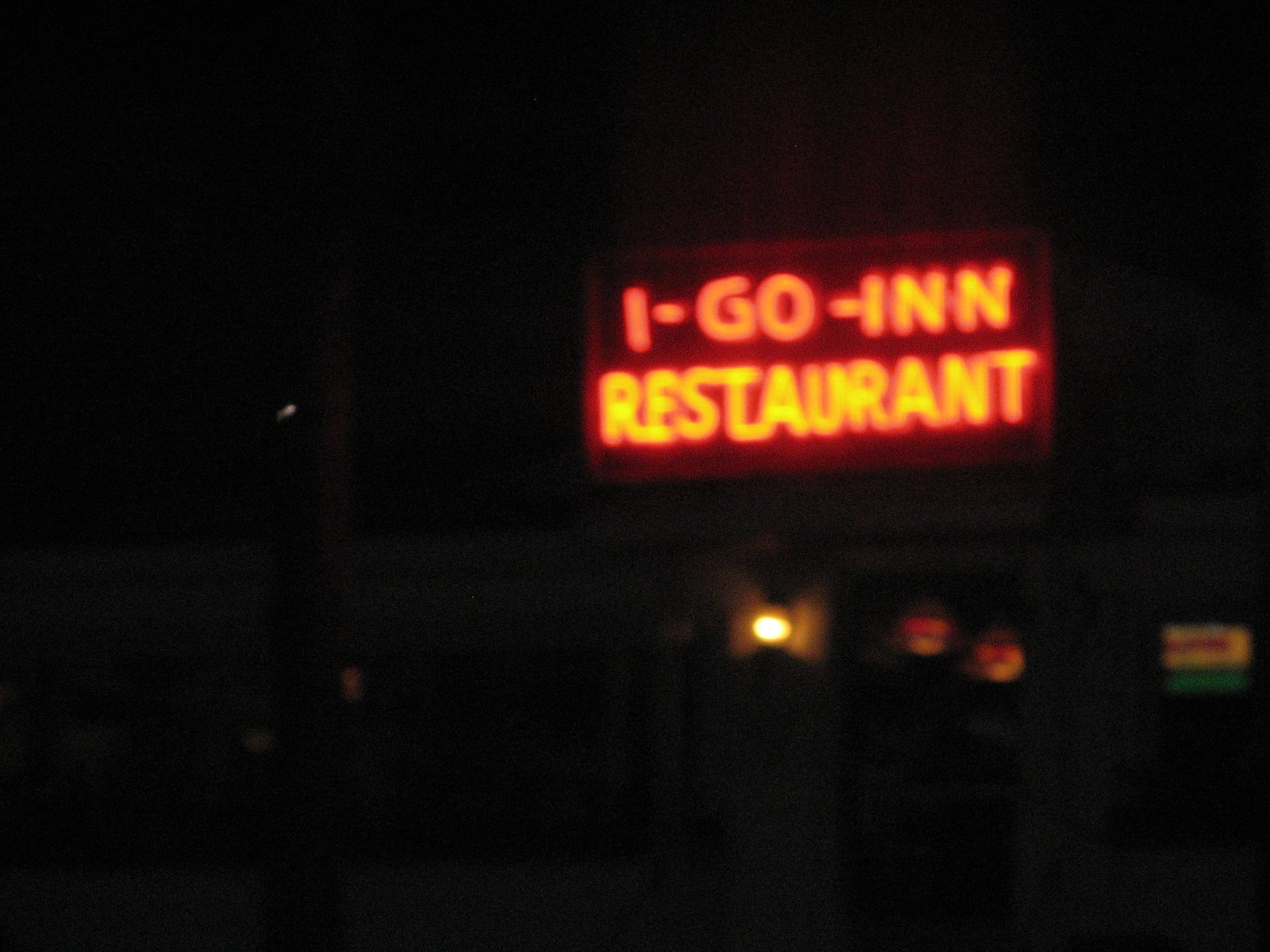In this nighttime photograph, darkness envelops the scene, creating a stark contrast with the vivid illumination from a striking neon sign. The sign, glowing with a reddish hue, boldly proclaims "I-GO-INN RESTAURANT" in all capital letters. Each letter is outlined in a bright yellow light, standing out against the blackness that surrounds them. Below the sign, the silhouette of the restaurant is visible, with faint lights glowing in its windows, hinting at activity inside despite the late hour. The faint outline suggests a cozy, welcoming establishment, illuminated just enough by the interior lights to offer a glimpse of its structure and inviting ambiance.